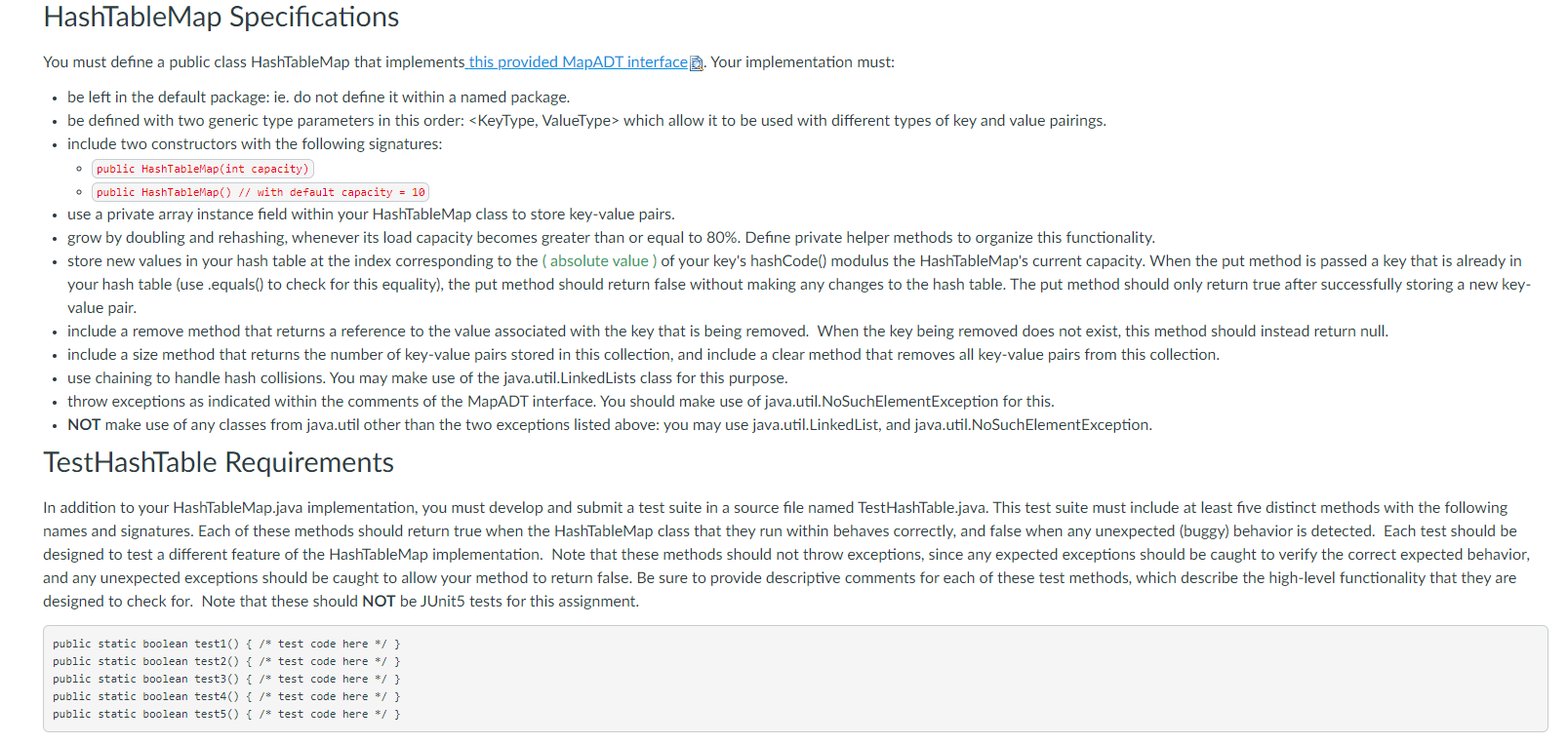The image displays detailed instructions for defining a Java class titled "HashtableMap" without a specified URL or website reference, indicated by the text on the left: "#HashtableMap specifications". Below this heading, in blue and underlined text, the instruction reads: "You must define a public class HashtableMap that implements the Map<K,V> interface."

The list of implementation requirements is presented in bullet points as follows:
- **Default Package Requirement:** The class must remain in the default package, meaning it should not be defined within any named package.
- **Generic Type Parameters:** The class should be defined with two generic type parameters in the following order: Key type (K) and Value type (V). This allows the class to be utilized with various types of key-value pairings.
- **Constructors:** Two constructors must be defined with the subsequent signatures:
  - `public HashtableMap(int capacity)` (highlighted in red)
  - `public HashtableMap()` (with a default capacity of 10, also highlighted in red)
- **Private Array Instance Field:** The class should use a private array instance field to store key-value pairs.

The instructions emphasize maintaining the class's location, ensuring flexibility through generic types, and stipulating specific constructors and storage mechanism.